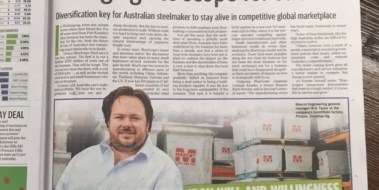The image is a photograph of a newspaper article. Although the heading is cut off, the visible content reveals the article is titled "Diversification Key for Australian Steelmakers to Stay Alive in Competitive Global Marketplace." The article focuses on strategies for Australian steelmakers to remain viable in a challenging industry. 

The newspaper is open, and on the left side opposite the article are what appear to be stock prices or various graphs depicting financial data.

Central to the article is a photograph of a man with brown hair, a beard, and a mustache. He has a sturdy build and is wearing a button-down white shirt. The man is superimposed in front of an image showing storage containers marked with a red "M" and some white lettering. In the upper corner of the photograph, there is black writing, likely providing additional details about the man and his relevance to the article.